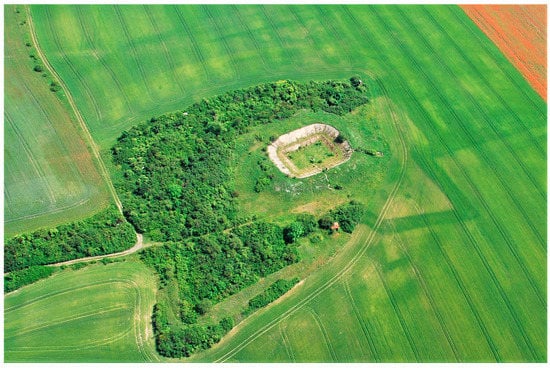This aerial photograph showcases a vast landscape dominated by lush green grass, carefully manicured into rows that stretch across the expanse, indicative of a well-maintained field. The image is brightly lit under sunny conditions, revealing fine details of the terrain.

In the center, there is a distinctive feature: a large, bowl-shaped depression resembling a small football field, though its exact nature remains uncertain. This depression, with its brown, rocky perimeter and green field within, adds an intriguing focal point to the image. Surrounding this central area is an assortment of dense trees, interspersed with various pathways and tire tracks, suggesting regular human activity.

In the upper right corner of the photograph, a contrasting patch of orange land, likely a field of crops, adds a splash of vibrant color against the predominant greenery. The image's perspective, possibly captured by a drone or plane from several hundred feet above, allows for a comprehensive view of this landscape, highlighting the blend of natural and cultivated elements seamlessly.